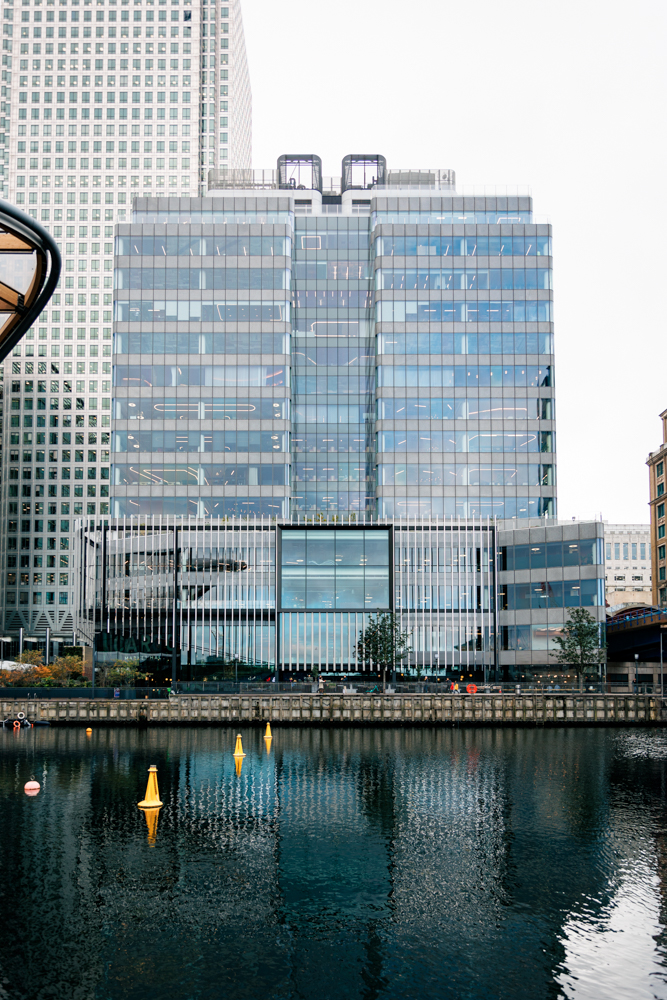In this photograph, we see an impressive cityscape prominently featuring a large, glass-fronted building set against an overcast gray sky. The building, which is symmetrical with a recessed middle section, boasts at least a dozen floors and is adorned with distinctive white bars along the first few levels, adding a stylized touch to its façade. This structure stands alongside a waterway, possibly a lake or a river, whose clear surface mirrors both the building and three small, pillar-like beacons or buoys situated in the water. Just beyond this impressive edifice lies a dock, and further in the background, to the left, looms an even taller skyscraper, likely a hotel, with numerous windows of its own. The reflective quality of the water captures the urban elegance, while a smattering of cars, trees, and people adds a dynamic, bustling ambiance to the scene.